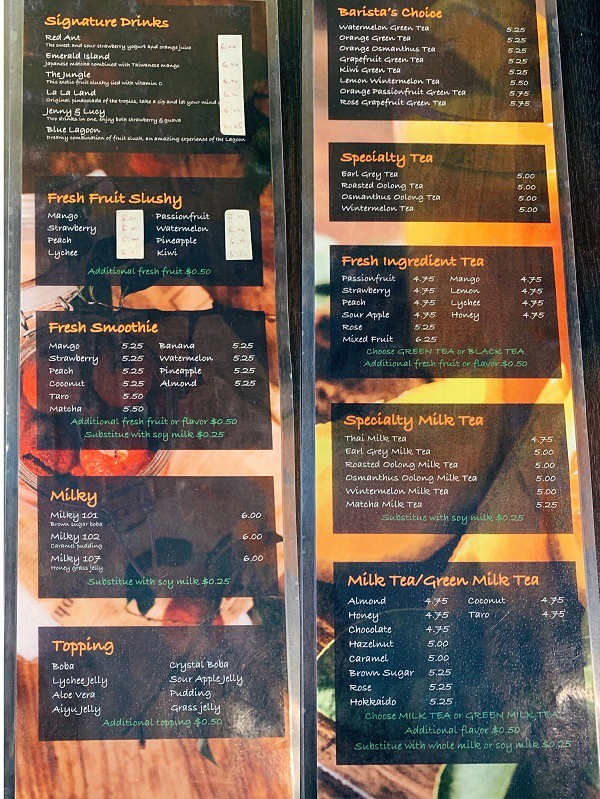This photograph captures a detailed image of a menu board within a boba tea or specialty tea shop. The menu is prominently displayed against the wall and consists of two panels, each framed in black with a dark background, enhancing the contrast and readability of the content. Illuminated by a light source entering from the bottom right corner, the menu is clearly visible. 

The left panel features sections titled "Signature Drinks," "Fresh Fruit Slushy," "Fresh Smoothie," and "Milky Topping." The background of this panel is adorned with vibrant fruit imagery, enhancing the fresh and fruity theme of the offerings. 

The right panel lists "Barista's Choice," "Speciality Tea," "Fresh Ingredient Tea," "Speciality Milk Tea," and varieties such as "Milk Tea" and "Green Milk Tea." This side also features a similar fruit-themed background, which blends harmoniously with the panel's content.

Both panels are set against a black backdrop, their black rims providing a polished, cohesive look. The fruits depicted in the background create a lively and inviting atmosphere, fitting for a place specializing in diverse tea-based beverages.